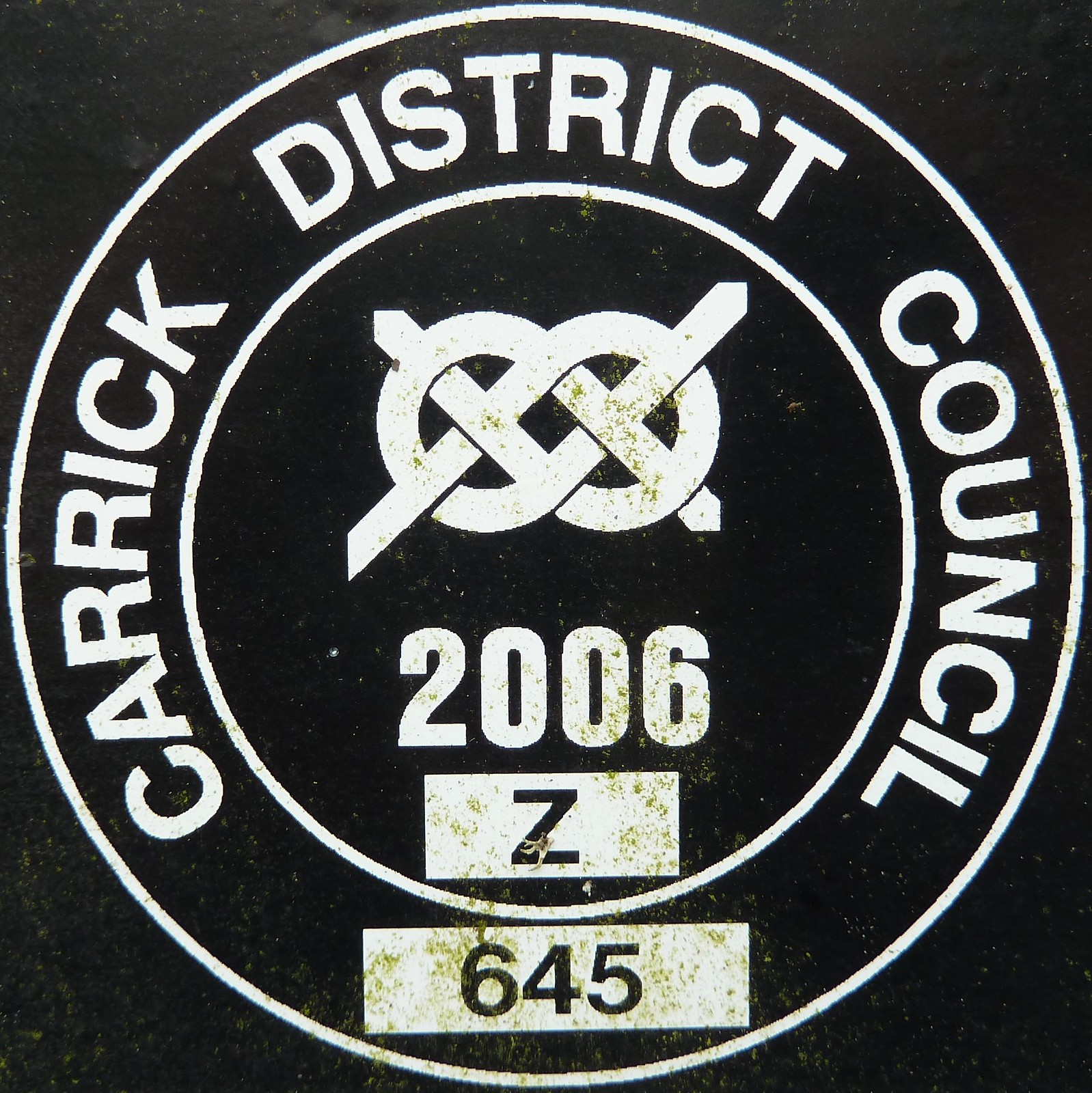The image displays a square black background with a central circular emblem outlined by two concentric white bands. The outermost band features the white uppercase text "CARRICK DISTRICT COUNCIL." Just below this text, also along the outer band, is a longer white rectangle containing the number "645" in black print. Within the inner circle, there is a distinctive emblem resembling a Celtic knot. Below this knot, the number "2006" is clearly printed, followed by a white rectangle containing a capital letter "Z." The overall design is simple yet detailed, primarily utilizing a monochromatic black and white color scheme for a striking visual contrast.